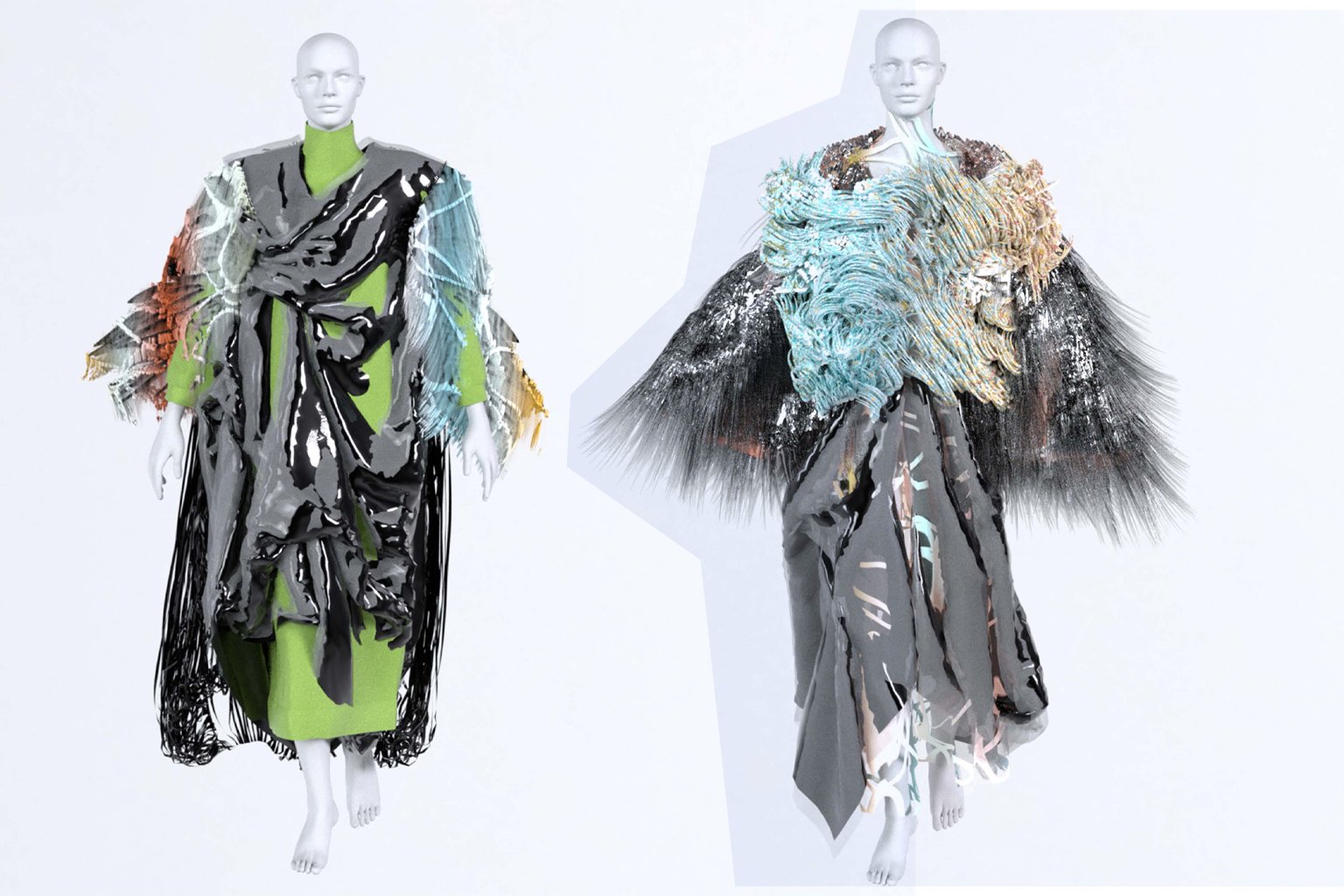The image is a computer-generated, landscape layout with an off-white background featuring two white mannequin models without hair or detailed facial expressions. The figure on the left is draped in an ensemble with a shiny, tar-like black texture. It wears a long-sleeved, green turtleneck dress extending to the ankles, adorned with a heavy, multicolored cloak incorporating shades of gray, white, blue, orange, and red, and decorated with blue feather-like accents. The mannequin on the right is clad in a voluminous gray poncho with blue and red designs. This figure also features a feathered black and white top, and its chest bears blue and orange details, completing the look with a combination of gray, black, turquoise, and cream hues.